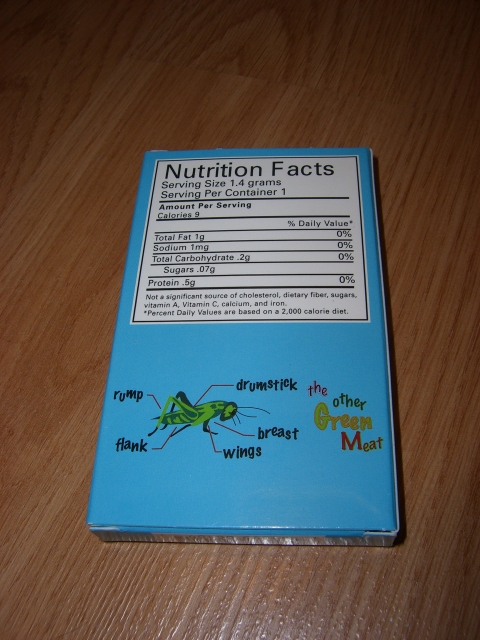This image displays the back of a small, light blue box, prominently featuring "Nutrition Facts" at the top. The nutrition label indicates that the serving size is 1.4 grams, with each serving containing 9 calories, and there is only one serving per container. The box also showcases an illustration of a cricket, with labeled parts such as "rump," "drumstick," "flank," "wings," and "breast," implying the consumption of crickets. It bears the caption, "The other green meats," suggesting a sustainable or eco-friendly protein source. The box is photographed resting on a wedding table.